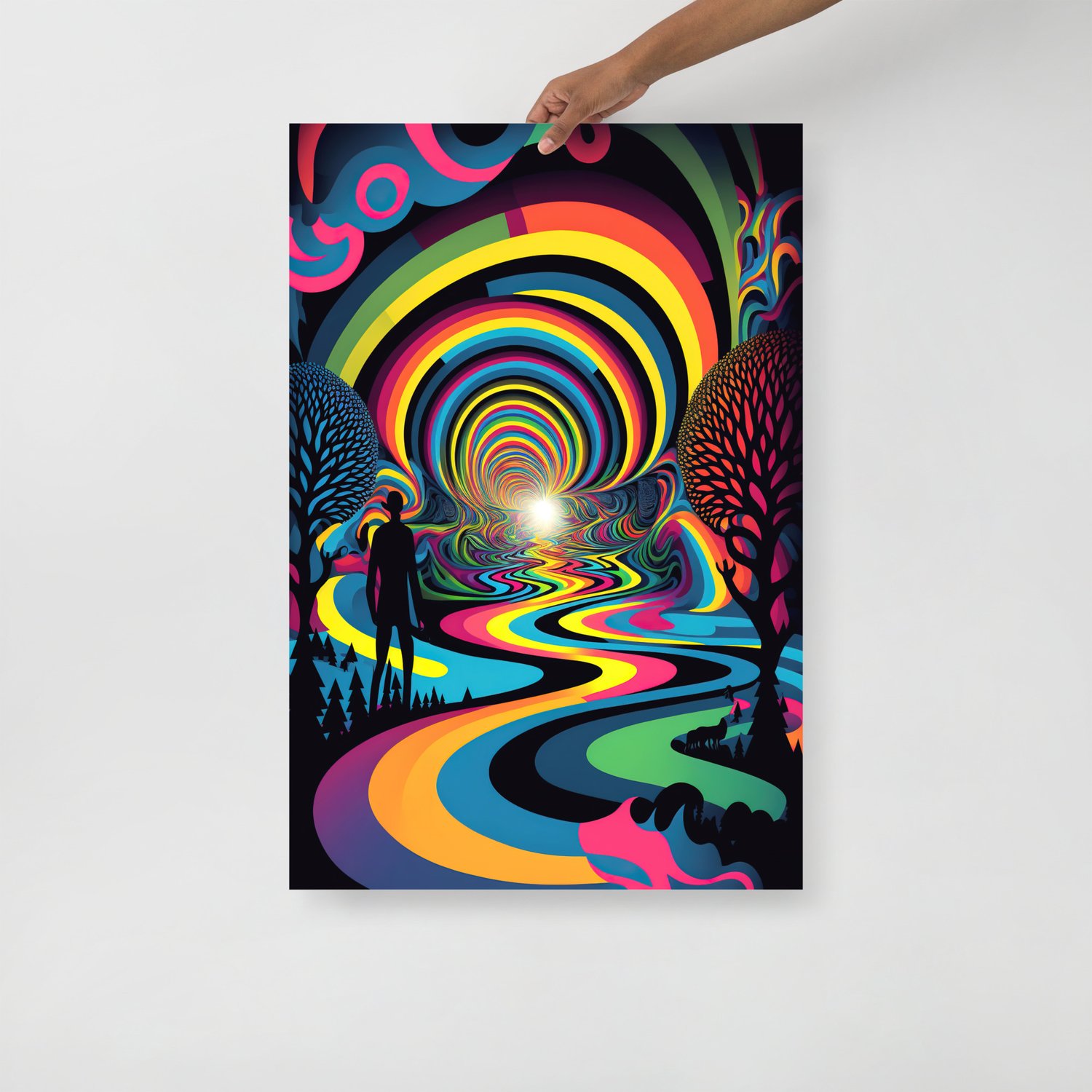A vibrant, poster-sized painting is displayed against a solid white wall, held up by a tan-skinned hand, visible from the wrist down to about half of the forearm, positioned at the top center of the image. The artwork bursts with neon and bright rainbow colors, creating a psychedelic effect. Dominating the image is a swirling, funnel-like tunnel composed of colors including green, orange, yellow, blue, purple, and red, creating a hypnotic visual. A twisted, colorful road extends from the tunnel, drawing the eye forward. Throughout the scene, various trees with red and blue leaves dot the landscape. A shadowy figure dressed in black attire and a hat walks along the path towards the mesmerizing spiral. The overall effect evokes a sense of surrealism and endless imagination, capturing a dreamlike journey that captivates the viewer's mind.